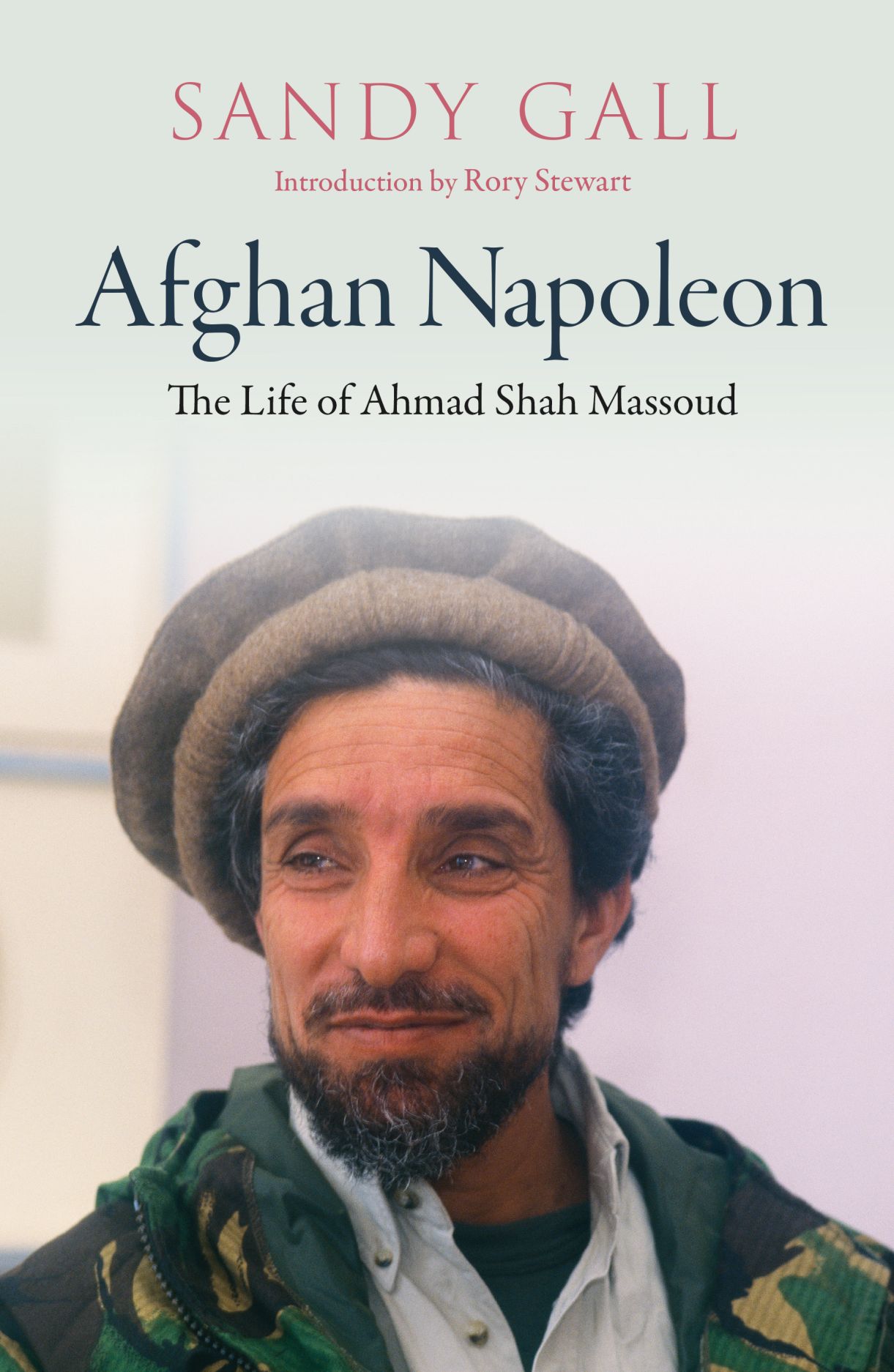The cover of the book "Afghan Napoleon: The Life of Ahmad Shah Massoud" by Sandy Gall, with an introduction by Rory Stewart, features a striking image of Ahmad Shah Massoud, a renowned Afghan warlord who sought to unify his nation. The title and author's name are prominently displayed in red text, with the introduction credited in smaller red letters. The main title appears in bold, dark black text, emphasized by the subtitle beneath it.

The cover art commands attention with its detailed portrayal of Massoud. He wears a distinctive brown hat, has dark, slightly graying hair, a beard, and bears smile lines and wrinkles around his eyes, adding a sense of wisdom and experience to his visage. Massoud is dressed in a camel jacket, which some may see as green with a camo print, over a white shirt and a black t-shirt. His contemplative gaze is directed to the left, suggesting a reflective mood.

This vivid and evocative cover places Massoud against a subtle, lightly colored background that may hint at buildings, but overall remains plain, ensuring that the focus remains on the subject of the biography.